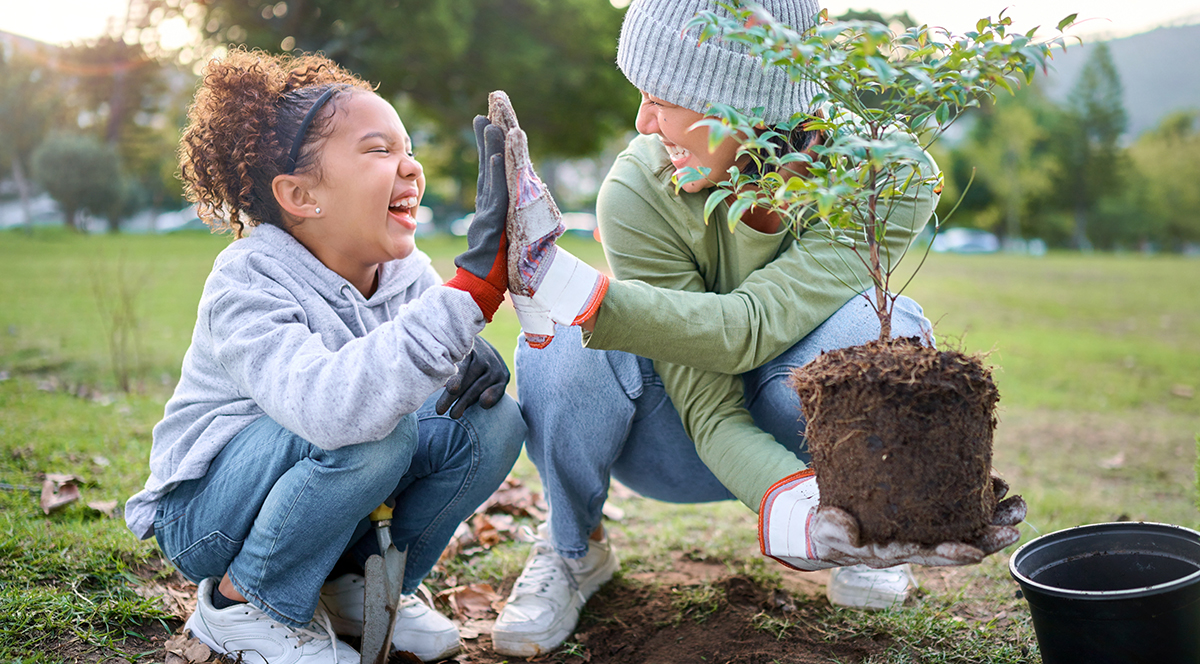In this vibrant and heartwarming photograph, a woman and a young girl, around 7 or 8 years old, are joyfully engaged in gardening in what appears to be a lush, green park. Centered in the image, both of them are squatting down, with the woman on the right and the girl on the left. They are captured in a delightful moment of laughter as they high-five each other, their faces beaming with joy and their eyes closed in the shared moment of happiness.

The little girl, adorned with a headband and earrings, sports curly brown hair styled in pigtails. She is wearing a gray hoodie, denim jeans, and white tennis shoes, with a small shovel in one hand and one hand up in a black and red gardening glove for the high-five. The woman, dressed in a green sweatshirt, denim pants, white tennis shoes, and colorful gloves, wears a dark gray beanie. Holding a large green plant that is ready to be replanted into a freshly dug hole, she shares this triumphant moment with the girl. The background showcases a serene park setting with out-of-focus trees, emphasizing the positive and nurturing atmosphere of their gardening adventure.